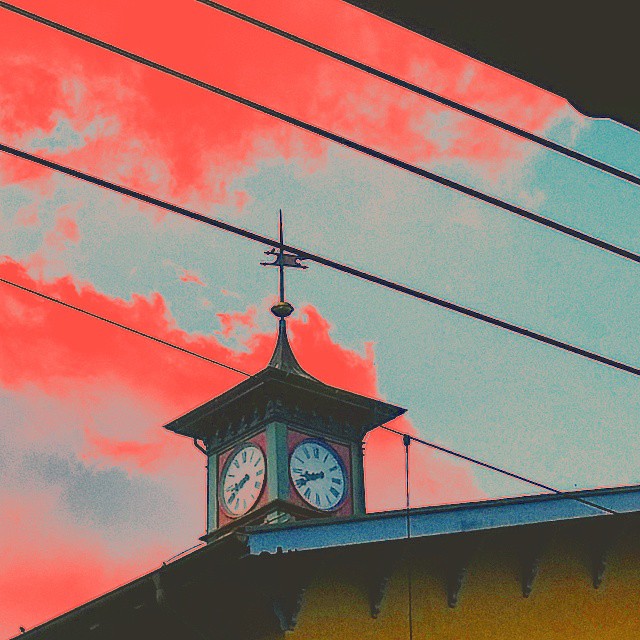A stylized image captures the dramatic beauty of a clock tower set against a vivid sky ablaze with pink and orange hues, suggesting the magic of either sunrise or sunset. The clock tower itself, a classical design capped with a pointed rooftop and crowned with a weather vane, stands as the foreground's focal point. Its muted colors contrast strikingly with the intense sky, highlighting its traditional elegance. The clock face, prominently displaying Roman numerals, exudes a timeless charm. Below the roofline, intricate woodwork showcases the meticulous architectural details. Adding a touch of modernity to the picturesque, old-fashioned scene are power lines that intersect the view, introducing a subtle, yet noticeable, blend of the past and present.